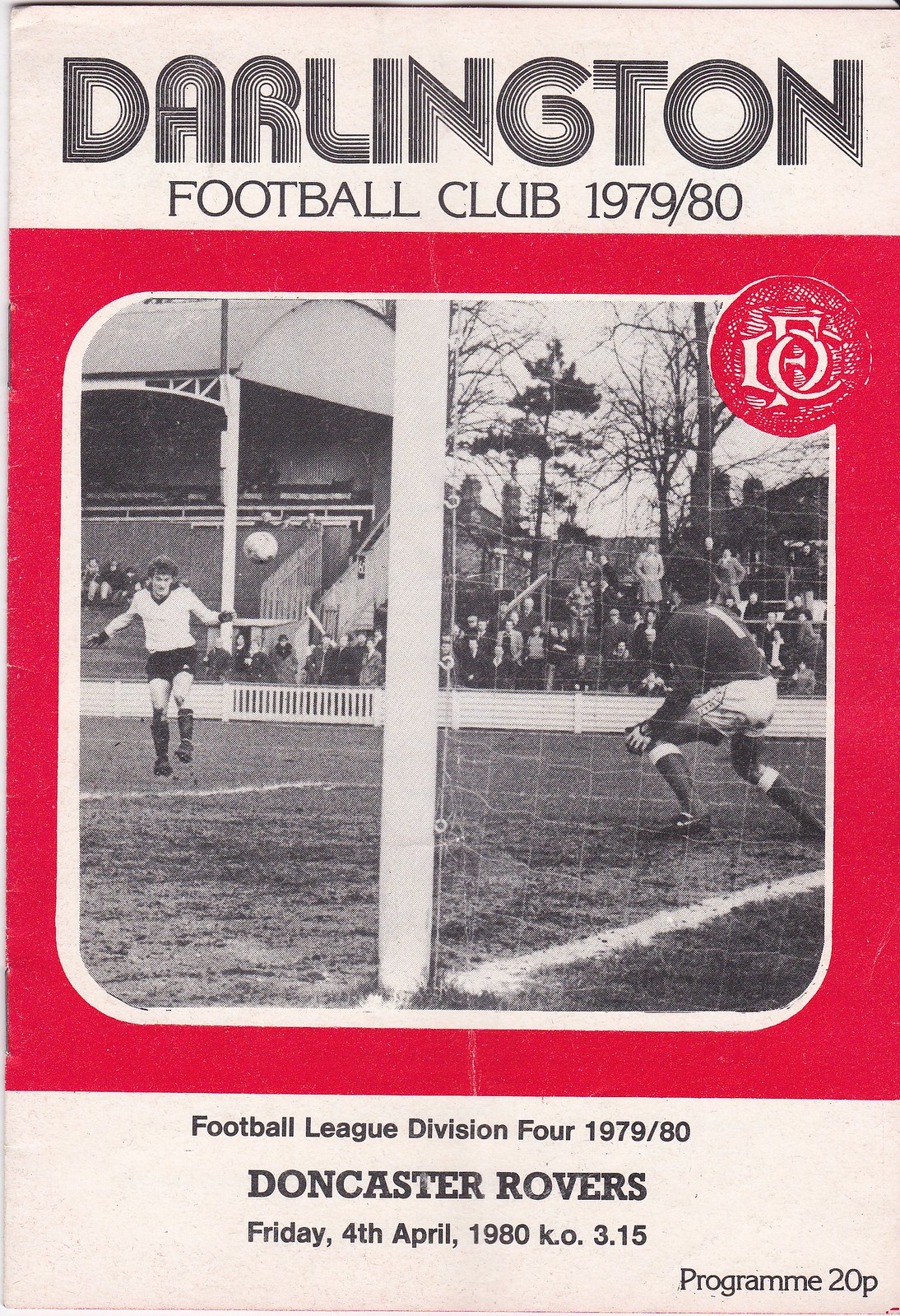The image depicts an old program booklet for Darlington Football Club from the 1979-1980 season. The program, which cost 20 pence, is designed with a red, black, and white color scheme. The title "Darlington Football Club 1979/80" is prominently displayed at the top against a white rectangular background with stylized black text. Below, there is a vivid red section holding a central black-and-white photograph framed by a red border with rounded corners. The photo captures dynamic soccer action: a player on the left kicking a ball towards the goal on the right, where a goalkeeper prepares to make a save. Separating the two black-and-white photos is a vertical white strip. The bottom section features more black text over a white background, detailing "Football League Division 4 1979-80" and specifics of a match against Doncaster Rovers on Friday, April 4, 1980, with a kickoff time of 3:15 PM (noted as K.O. 3:15).